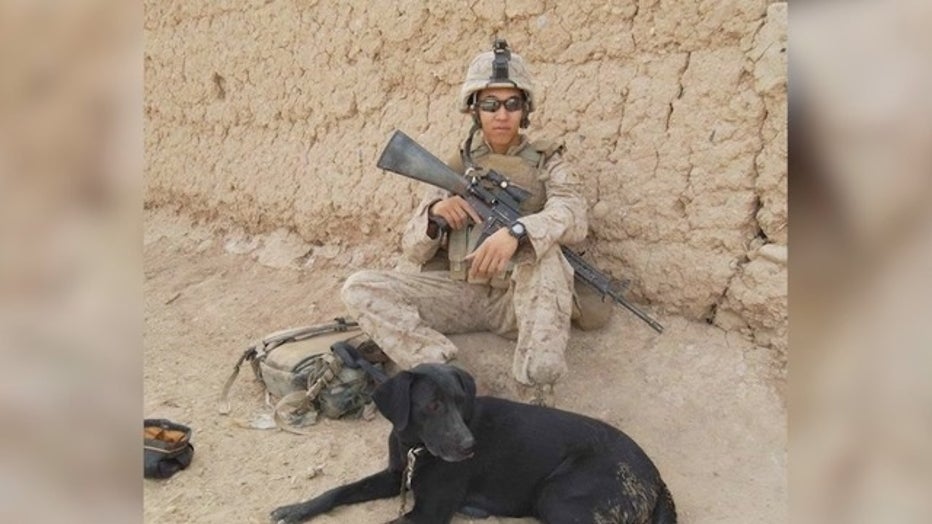The image captures a soldier seated against a heavily cracked, dried mud wall in a desolate, desert-like environment, indicative of the Middle East. The soldier, clad in tan-colored combat fatigues and body armor with pouches for rifle magazines, holds an automatic rifle equipped with a scope across his lap. Tan boots, scuffed and sandy, complement his attire. Next to him, on his left side, a tan backpack nestles under his leg, and a smaller black bag lies nearby. In front of the soldier, a black Labrador retriever is lying down, a leash connecting its collar to the soldier’s hand, suggesting companionship. The overall scene is bathed in muted tones of tan, black, and hints of flesh color, rendering a somber, yet intimate portrayal of a moment from the soldier’s deployment, perhaps captured from a video due to the blurred edges surrounding the frame.